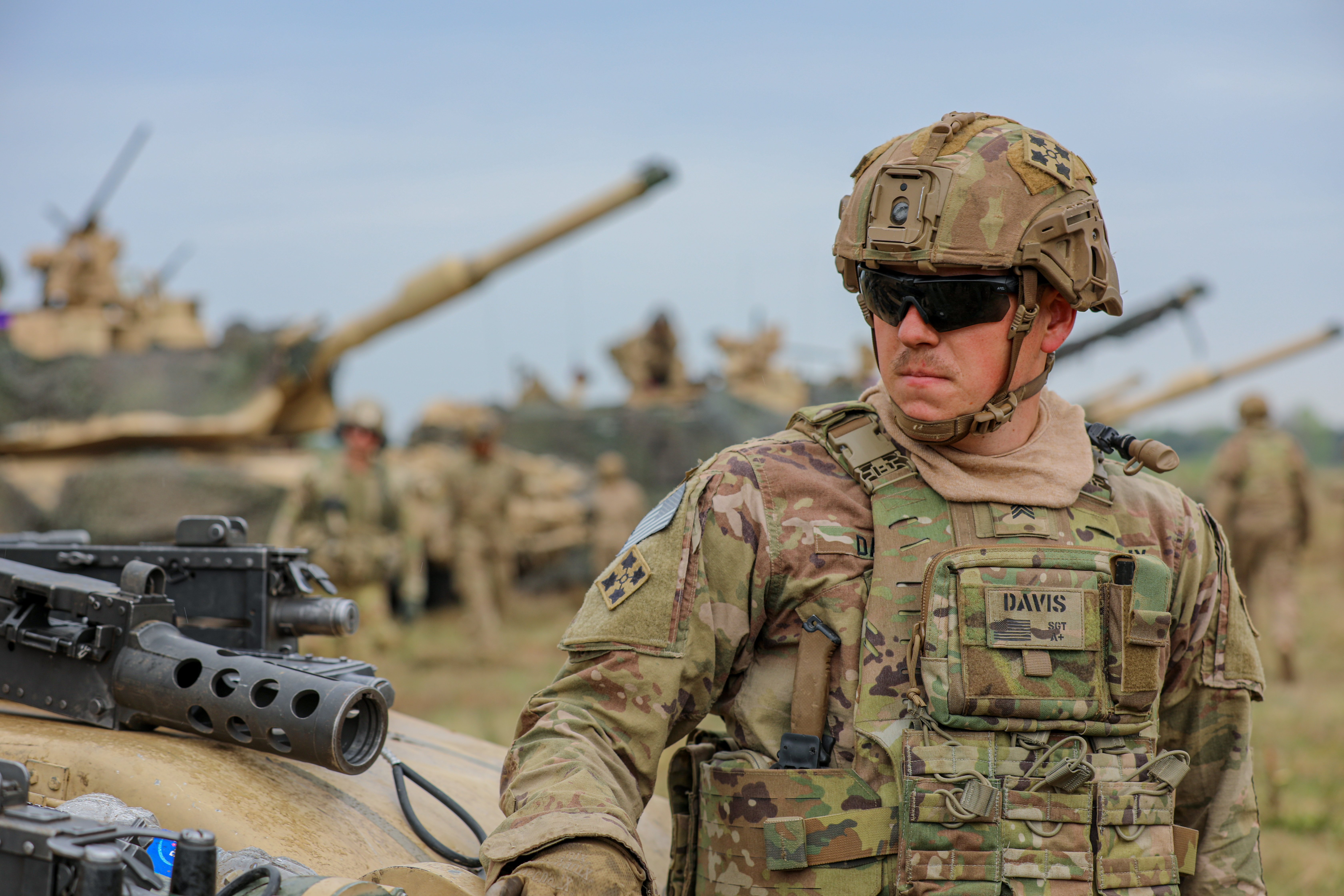In this detailed image, we see an army soldier named Davis prominently positioned on the right side. Davis, identifiable by his name tag, is dressed in full military attire consisting of camouflage patterns in shades of green, brown, and black. He wears a helmet secured with a chin strap and sports black sunglasses, with a hint of a peach fuzz mustache visible on his white skin. His outfit and helmet are adorned with typical military camouflage, featuring a mix of dark greens and browns. To Davis's left, the black barrel of a heavy-duty gun with a perforated muzzle is visible, possibly part of a tank. In the background, slightly out of focus, are additional military personnel similarly dressed in camouflage, as well as several tanks. The background is framed by a sky that is either a deepening dusk or early morning blue, adding a serene contrast to the intense military scene.